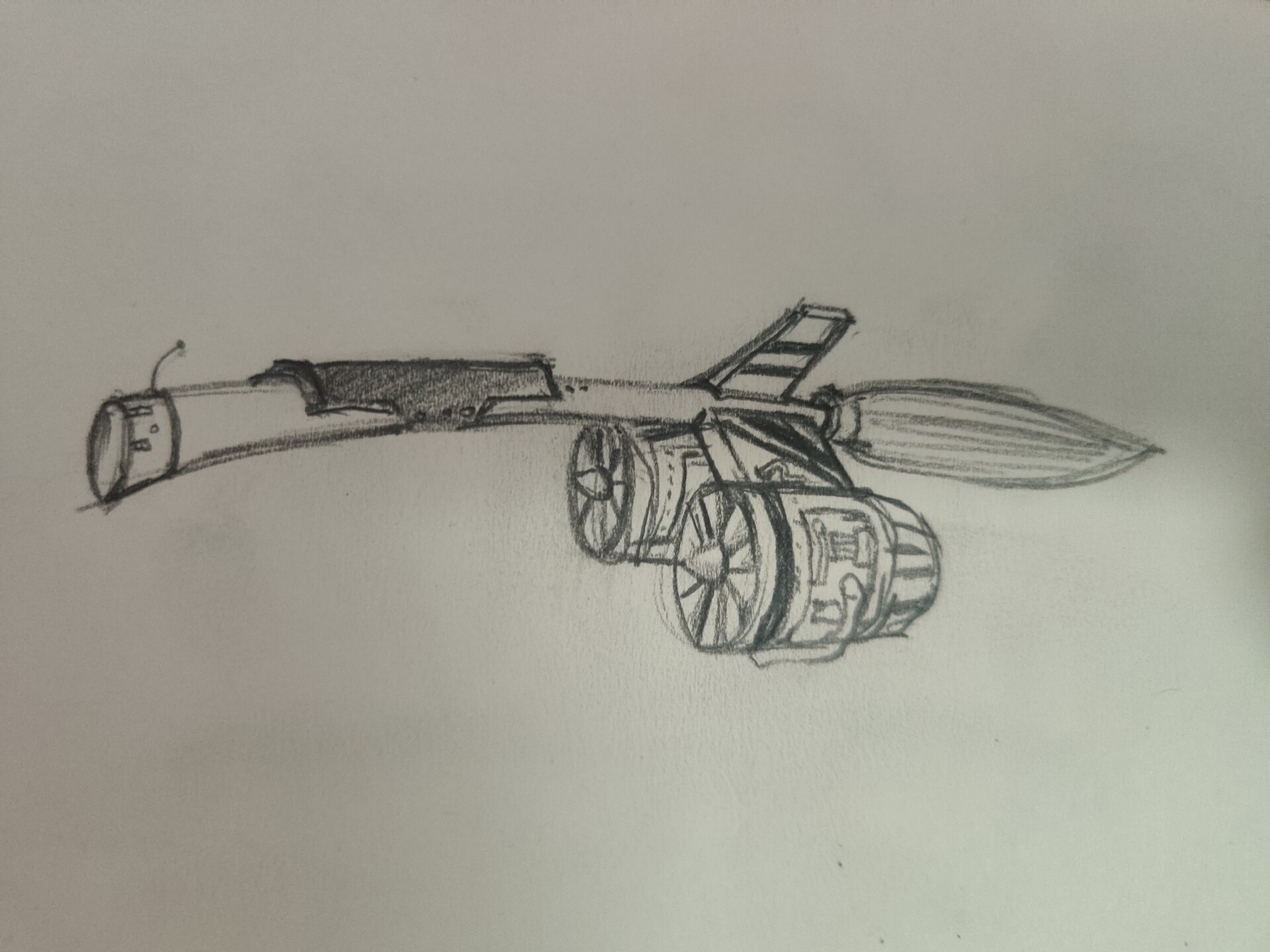The image is a highly detailed, pencil sketch of a steampunk-inspired rocket-like broomstick. This long, intricate broomstick features multiple triangular-shaped fins at the bottom, each adorned with large, circular jet propeller engines complete with front fans, cone shapes, and side pipes. The broomstick has a detailed saddle located midway up the shaft, above the motor canisters, and a small antenna at the top, complemented by what appears to be a metal plate. The broom's bristles are meticulously layered, adding to the elaborate design. The entire sketch is set against a white or whitish-gray background, showcasing the remarkable intricacy and craftsmanship of the drawing.